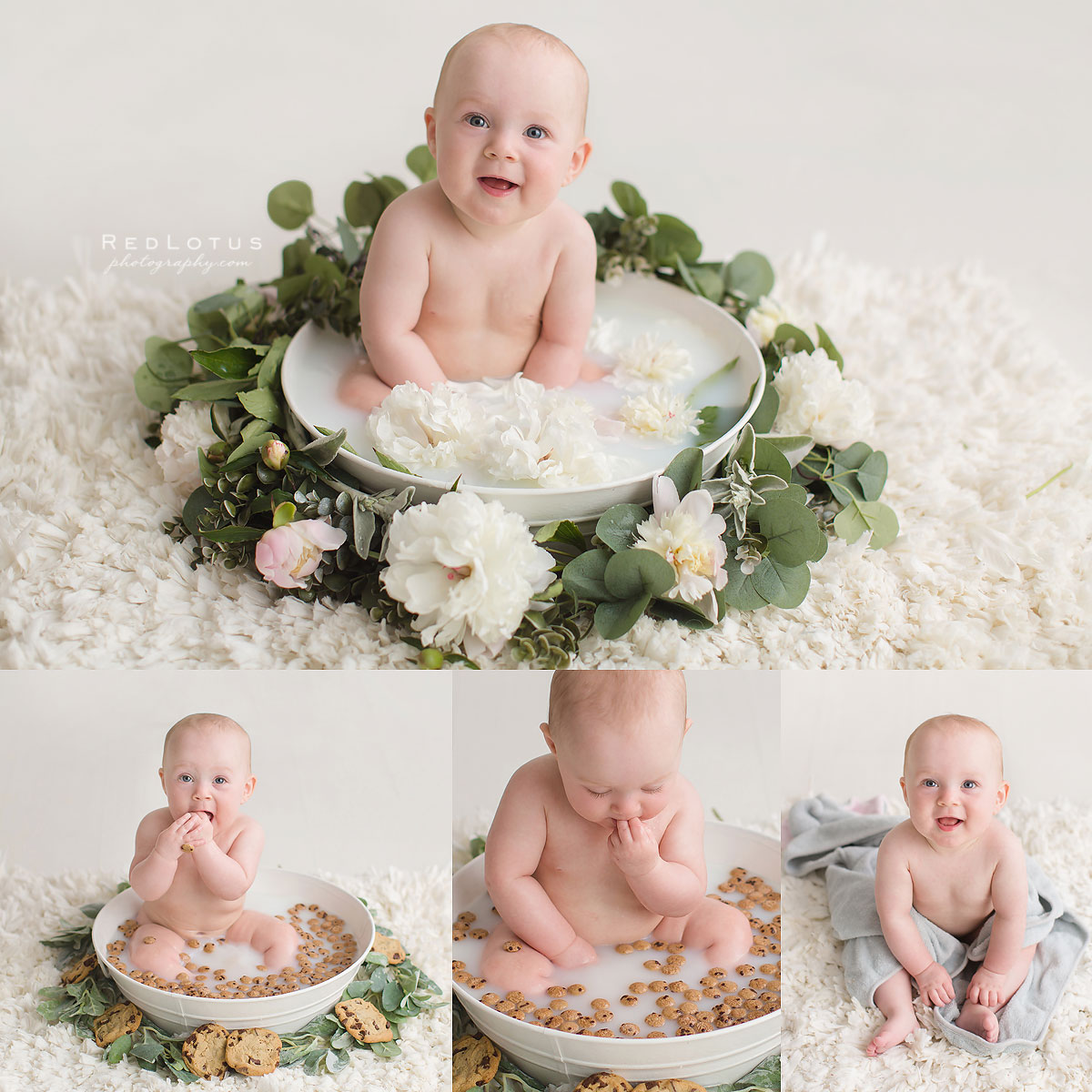This image set, presumably titled by RedLotusPhotography.com, features an adorable baby photo shoot comprising four distinct panels. The top panel, the largest, showcases a charming white baby with dark eyes sitting in a bowl filled with milky water, adorned with floating white flowers and a garland of green leaves and flowers around the bowl's edge. This panel also includes a pink flower amidst the decorative garland and is set against a fluffy white rug.

The bottom section consists of three smaller photos aligned horizontally. The first of these repeats the milk bath scene but replaces the flowers with cookie crisps floating in the milky water and chocolate chip cookies integrated into the leafy garland. The baby is depicted eating one of the cookies. The middle photo is an up-close shot of the baby enjoying the cookies. In the final image, the baby is seated on the soft white rug, wrapped in a cozy gray towel, and smiling up at the camera, creating a warm and delightful series of snapshots.